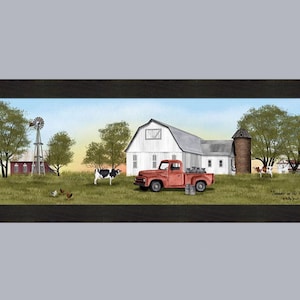This image appears to be a small, horizontal, colored pencil drawing inside a gray box. It features a rural farm scene with a prominent old-style red pickup truck parked on vibrant green grass. The truck is centered in front of a large, white barn with a brownish silo extending from its right side. To the left of the truck stands a black and white cow. Further left, closer to the background, there's a windmill and a red outbuilding with a white roof. Three chickens are scattered near the cow, adding to the picturesque farm setting. The scene is framed by lush green trees on both sides. The sky transitions from baby blue to yellow, hinting at either sunrise or sunset, with a reddish glow peeking from the far distance.